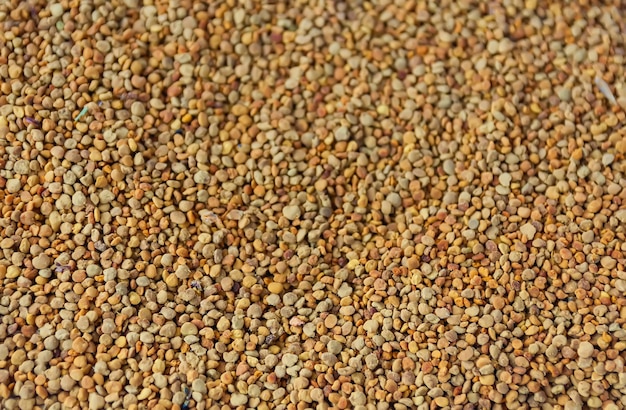This close-up, rectangular photograph captures a spread of small pebbles, reminiscent of those found at a gravel pit or construction site. The pebbles, predominantly rounded and smooth, range in size from that of a dime to a nickel. Their color palette encompasses various earthy hues, primarily sandy tan, with accents of brown, orange, yellow, and cream. The largest pebbles are cream-colored while the smaller ones exhibit shades of reddish-yellow to yellow-orange. Despite a slight blur at the top, the image is a clear depiction of numerous tiny stones, presenting a textural and visually diverse mixture. This photograph could serve as a naturalistic background or wallpaper, evoking a sense of organic, grounded simplicity.